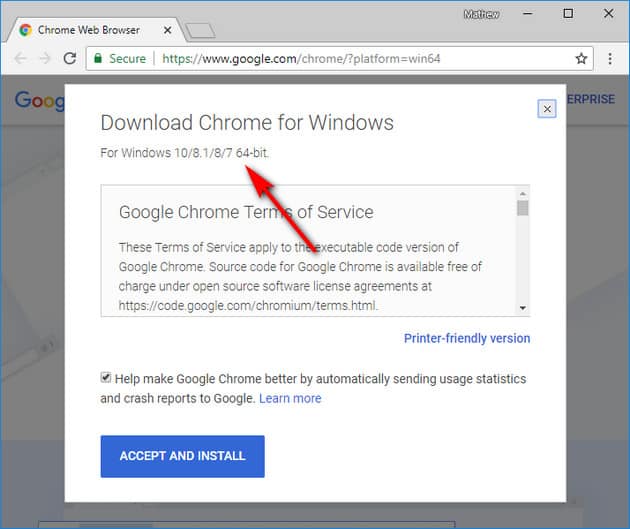Here's a detailed descriptive caption for the image:

---
This image is a detailed screenshot from the Google Chrome web browser. The user, identified as Matthew (spelled with one 'T'), has the Google homepage open in the background. Dominating the foreground is a prominent white dialogue box with the heading in dark grey text that reads, "Download Chrome for Windows." Just below, it specifies compatibility details in smaller font: "For Windows 10/8.1/8/7 64-bit."

Under these instructions, a comprehensive description of the Google Chrome terms of service is displayed. The text explains the terms' applicability to the executable code version of Google Chrome and mentions the availability of the source code under Open Source Software License Agreements. An address link is provided: [https://code.google.com/chromium/terms.html](https://code.google.com/chromium/terms.html). Additionally, there's an option for a printer-friendly version of the terms indicated in blue text.

A red arrow, drawn from the terms of service paragraph, points towards the operating systems compatibility information. Below the terms, there is a checkbox that is checked. The label beside the checkbox states, "Help make Google Chrome better by automatically sending usage statistics and crash reports to Google," followed by a "Learn More" link in blue. Towards the bottom of the window, there is a white tab with the text "Accept and Install," which is the call-to-action button to proceed with the installation process.
---